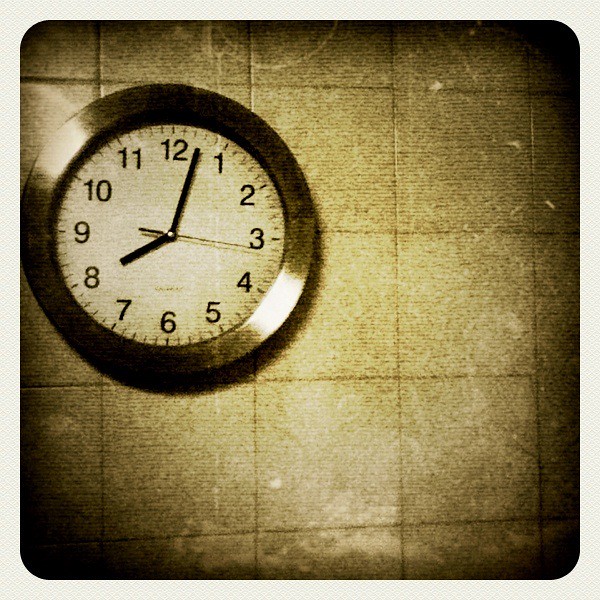This sepia-toned, square artistic photograph, potentially altered in Photoshop for an enhanced vintage feel, features a round clock prominently positioned at the left center against a uniformly tiled wall. The grainy texture of the background, evocative of an old film strip, adds to the nostalgic atmosphere. The clock displays the time as approximately 8:02, with a notable shine reflecting over the 10 o'clock position and below the 4 o'clock position, suggesting the presence of a light source. The clock's hands – minute, hour, and second – are all black, contrasting sharply with its face. The composition is subtly bordered by a square with rounded corners and a delicate white edge, framing the timeless scene and enhancing its antiquated charm.